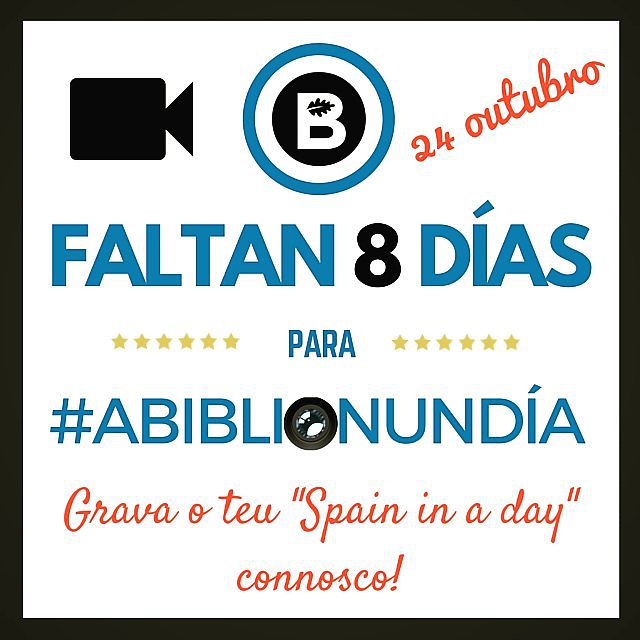This photograph features an advertisement for a local Spanish event, possibly in Spain. The design is bordered with a black padded outline, providing a bold frame for the content. In the upper left corner, there's a black logo resembling a camcorder, indicative of a focus on filming or recording. The top center displays a blue circle with a white letter 'B', adorned with a leaf motif at the upper segment of the letter. The text within the advertisement, written in Spanish, announces a countdown to the event: "24 Outubro" (24th of October), followed by "Faltan 8 días para" (8 days remaining until). Below this, a hashtag "#ABIBLIONUNDIA" and the phrase "Grava o teu Spain in a Day Connosco!" (Record your Spain in a Day with us!) emphasize the participatory nature of the event, inviting the audience to engage. This comprehensive advertisement clearly aims to attract local attention to the impending event, leveraging visual and textual elements to create a cohesive and compelling promotional piece.